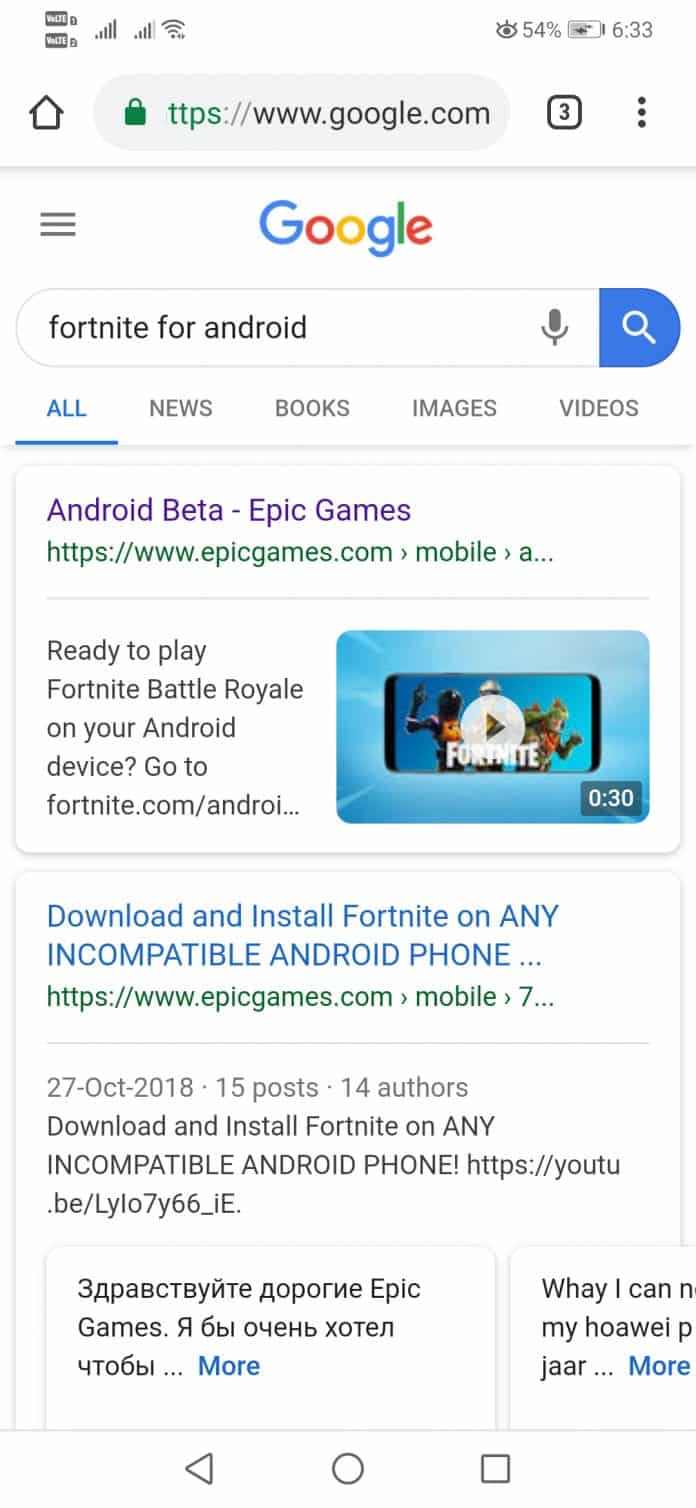The image displays a smartphone screenshot with the URL box at the top showing "google.com". The battery indicator shows 54% and the time is 6:33. Directly below the URL box is the Google logo in its signature multicolored letters. Beneath the logo, a search bar displays the query "fortnite for Android" and features both a microphone icon and a magnifying glass icon. Below the search bar, tabs labeled "All," "News," "Books," "Images," and "Video" are visible. 

Further down, there's a highlighted search result titled "Android Beta - Epic Games" from epicgames.com. The description reads, "Ready to play Fortnite Battle Royale on your Android device? Go to fortnite.com/android." This is followed by a prompt to download and install Fortnite on incompatible Android phones, dated "27 October 2018," and referencing "15 posts 14 authors." The lower part of the screenshot includes additional text, which is written in Cyrillic script.